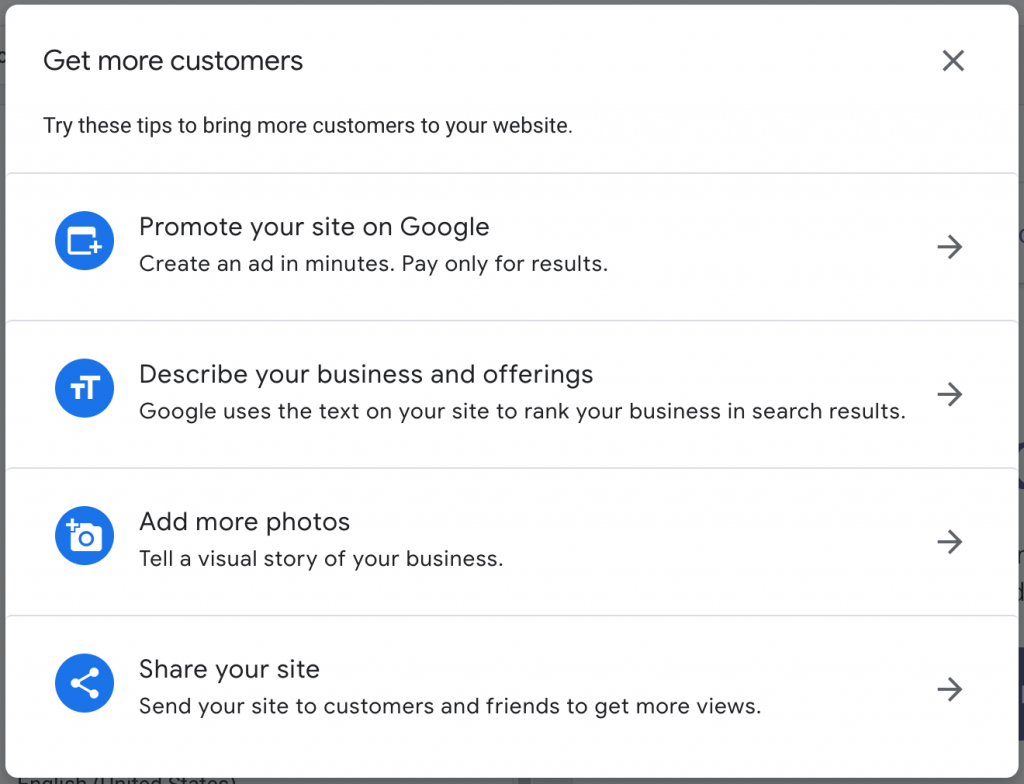The image is a screenshot of a promotional message aimed at helping businesses attract more customers to their websites. The central message, written in bold black text, reads: "Get more customers." To the right of this text is an 'X' button to close the message. Below the main message, there's a supportive statement: "Try these tips to bring more customers to your website."

The tips are presented in four distinct rectangular boxes, each accompanied by a blue circle with different icons:

1. **First Box:** Features a blue circle with a plus sign inside. The text in this box encourages businesses to "Promote your site on Google, create an ad in minutes, pay only for results." This box includes a gray arrow pointing right, suggesting additional information or steps.

2. **Second Box:** Displays a blue circle with two 'T' letters, one larger than the other, in white. This section advises, "Describe your business and offerings. Google uses the text on your site to rank your business in search results." Another gray arrow indicates more details are available.

3. **Third Box:** Shows a blue circle with a camera icon and a plus sign. The tip here is to "Add more photos, tell a visual story of your business," coupled with a right-pointing arrow for further actions.

4. **Fourth Box:** Contains a blue circle with an icon signifying sharing. It prompts users to "Share your site, send your site to customers."

Each section is designed to guide the user through different strategies to enhance their online presence and drive more traffic to their website.